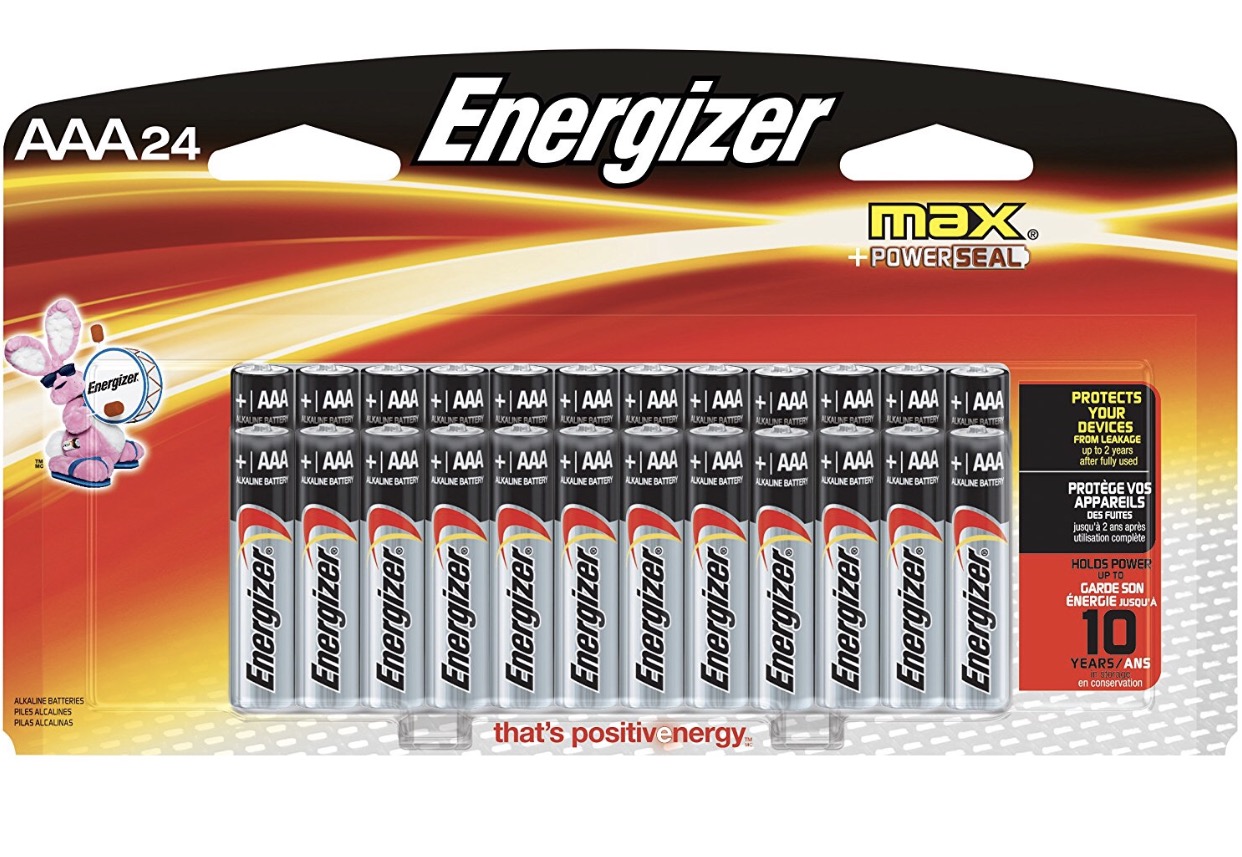This product photo showcases a 24-pack of AAA Energizer Max Plus PowerSeal batteries against a sleek black background. Dominating the upper portion of the packaging is a vibrant energy line gradient, blending red, yellow, and orange hues into flowing ribbon-like patterns. At the very bottom, this energetic display subtly transitions into a white and gray grid.

To the left of the package, roughly a couple of inches from the top, sits the iconic pink Energizer Bunny, instantly recognizable and symbolizing enduring power. The topmost section prominently displays "AAA 24," clearly indicating the product type and quantity.

The batteries are securely encased in a clear plastic blister pack, revealing their silver bodies and black tips. Each battery is marked with the Energizer logo, along with designations for "AAA" and "Alkaline Batteries."

To the right side of the packaging, there's an informative box detailing the product's unique features. It states, "This protects your devices from leakage up to two years after fully used," with a similar statement in French nearby. Additionally, the packaging boasts that these batteries "hold power up to 10 years," again accompanied by translations in multiple languages, underscoring its global appeal and reliability.